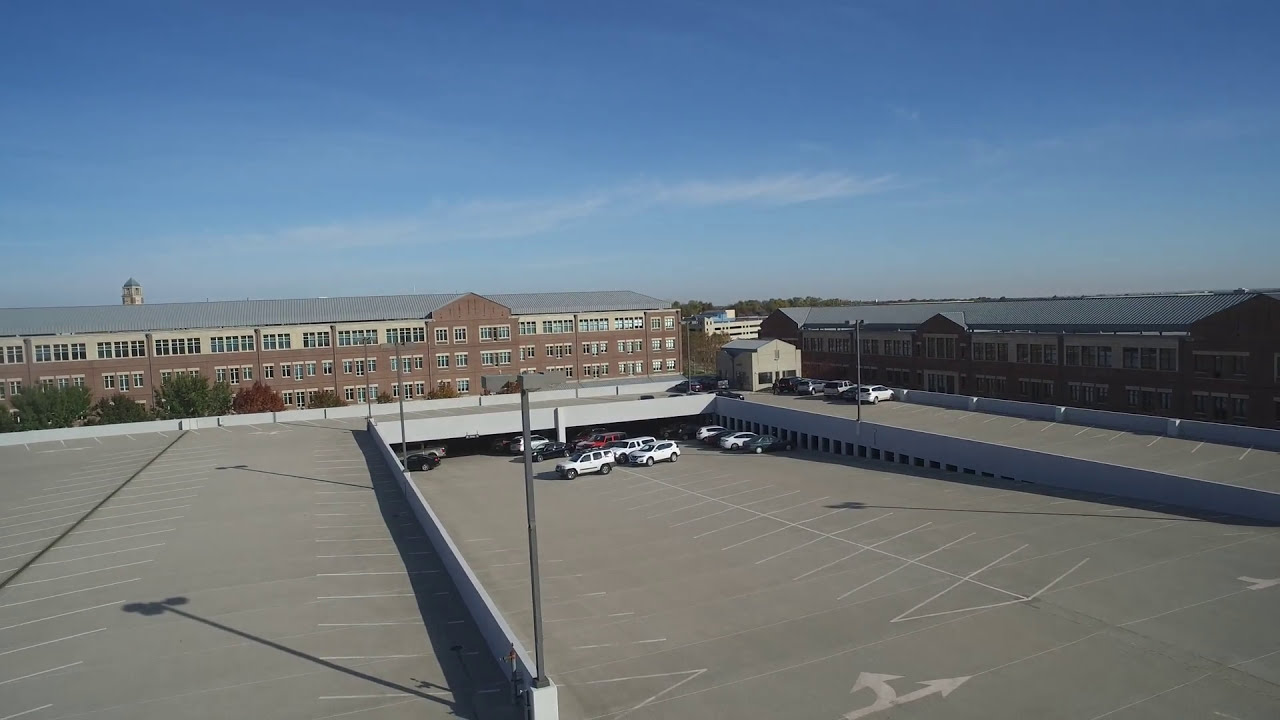The photograph captures a crisp, clear view of the rooftop of a parking garage on a sunny day with a nearly cloudless, light blue sky. The parking lot, which is seen from an elevated or drone perspective, features several empty spaces, with just a few vehicles—mostly white SUVs and a truck—parked in the central section. An arrow painted on the pavement directs traffic to the right and then curves towards the back of the image. To the right, a connecting section links to another part of the parking deck where four more vehicles are parked. In the background, a wide, red-brick building extends across the horizon, its purpose indistinct, possibly residential or commercial. Another similar brick building sits on the right, partially obscured by shadows. The scene is framed in a landscape orientation and showcases a realistic, photographic representational style.